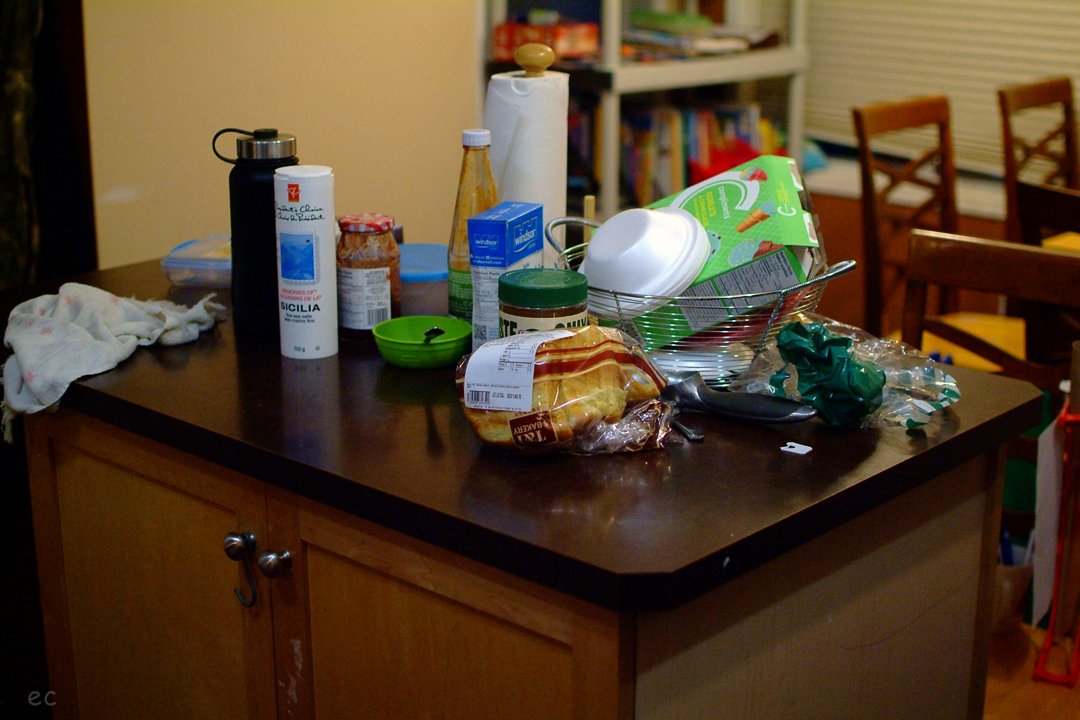The image showcases a lively activity space, possibly a playroom or an extension of a kitchen. Centrally, there is a dresser repurposed as a small island table, laden with an array of items hinting at meal preparation. The table holds bread, salt, jelly, a water bottle, a sauce container, styrofoam bowls, and a green snack box with white lettering. Among these, a paper towel roll stands on a wooden holder, and a clear glass Tupperware with a blue trim sits nearby. A green bowl with a spoon in it and a plastic bread wrapper suggest a mealtime setting.

To the right of the makeshift table, brown chairs with yellow cushions are arranged, likely for seating during the meal. Behind these chairs stands a white stackable shelf filled with various items, possibly books or other small objects, adding to the room's eclectic and functional vibe. The scene overall conveys the hum of an active household preparing for lunch or dinner.